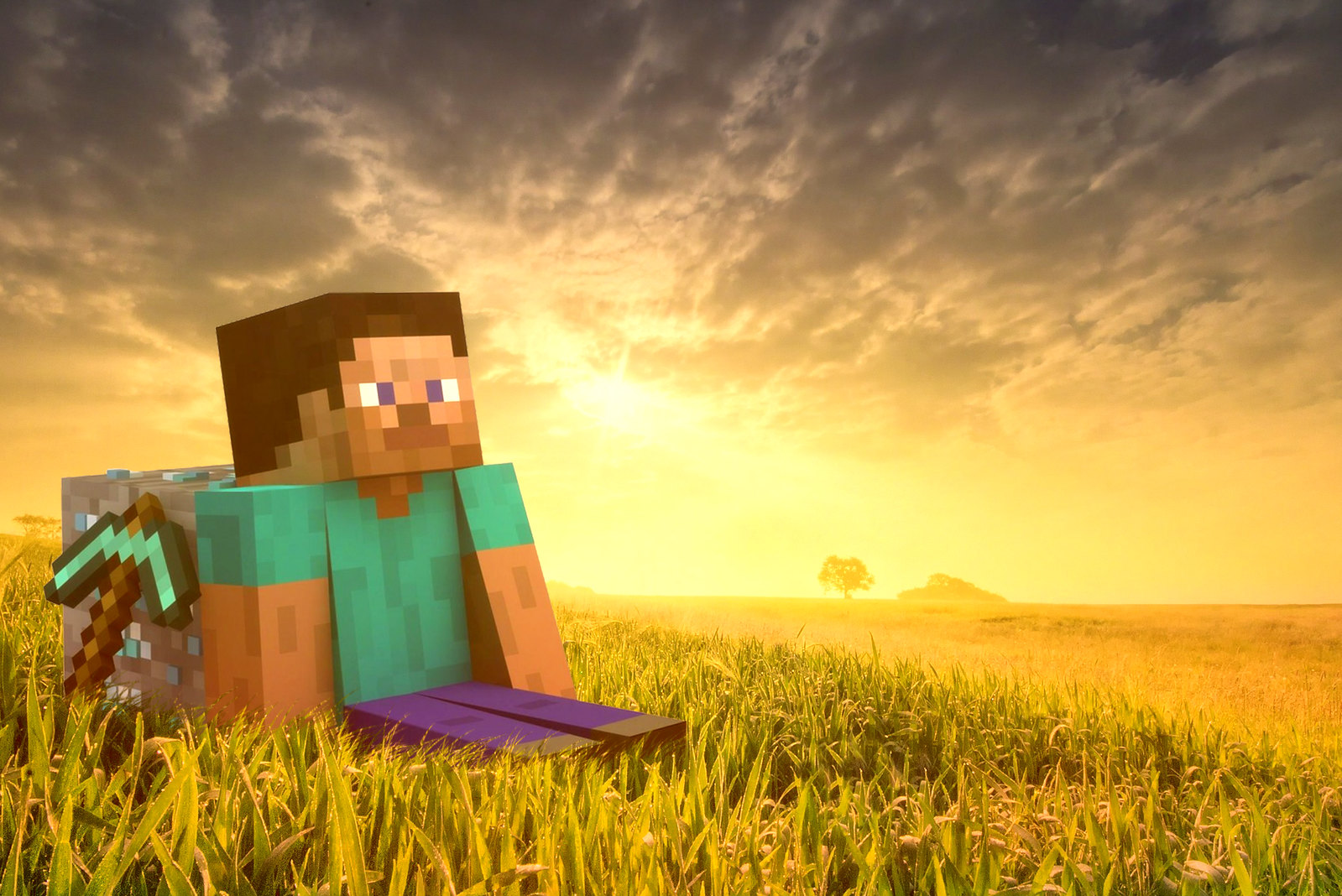In the golden light of dusk, a picturesque scene unfolds in a grassy meadow beneath a cloudy sky aglow with the sun's hazy radiance. Puffs of clouds scatter across the horizon, casting an ethereal yellow hue across the entire landscape, accentuating the single tree and distant mountain that frame the background. Nestled to the left in the foreground sits a heavily pixelated, boxy figure—reminiscent of the iconic Minecraft character, Steve. This 3D avatar, with a square head of brown hair and face of tan pixels, sports a teal short-sleeved shirt, purple pants, and brown shoes. His blocky arms and legs, partly accented with green and orange hues, extend straight out as he sits in the realistic grass. A stack of boxes lies behind him, along with a blocky object resembling a tree, identifiable by its brown trunk and green zigzag top. Another object, possibly a pickaxe, rests across his back, completing this surreal blend of virtual and natural worlds.